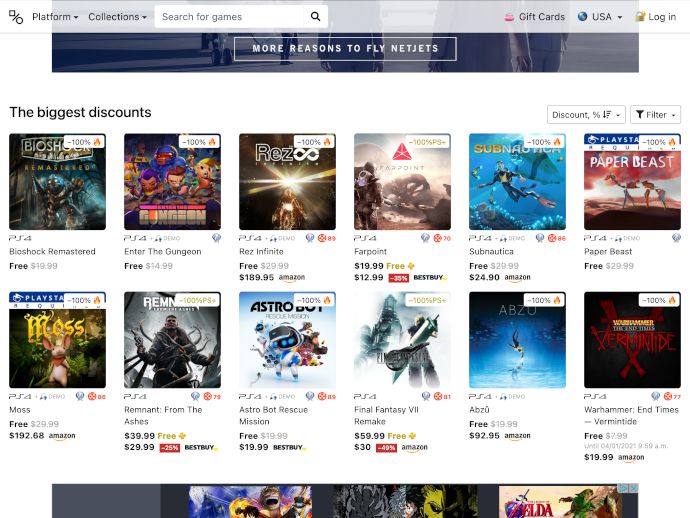In this image, we see a section of a video game platform interface. At the top, there is a search bar labeled "Search for games." Below the search bar, an advertisement banner reads "More Reasons to Fly NetJets," although it is not clear whether this ad directly relates to the games displayed.

The games are presented in two full rows, each containing six games, for a total of twelve visible titles. Additionally, below these rows, there is a partial view of three more games. The majority of the displayed games fall under the fighting genre or similar action-packed categories. 

Specifically, the games visible include "Bioshock Remastered," "Enter the Gungeon," "Rez Infinite," "Farpoint," "Subnautica," "Paper Beast," "Moss," "Remnant: From the Ashes," "Astro Bot Rescue Mission," "Final Fantasy VII Remake," and "Warhammer." Most titles are noted to be playable on the PS4 and are marked as free, except for "Farpoint," which appears to have conflicting labels indicating both a free status and a certain percentage discount.